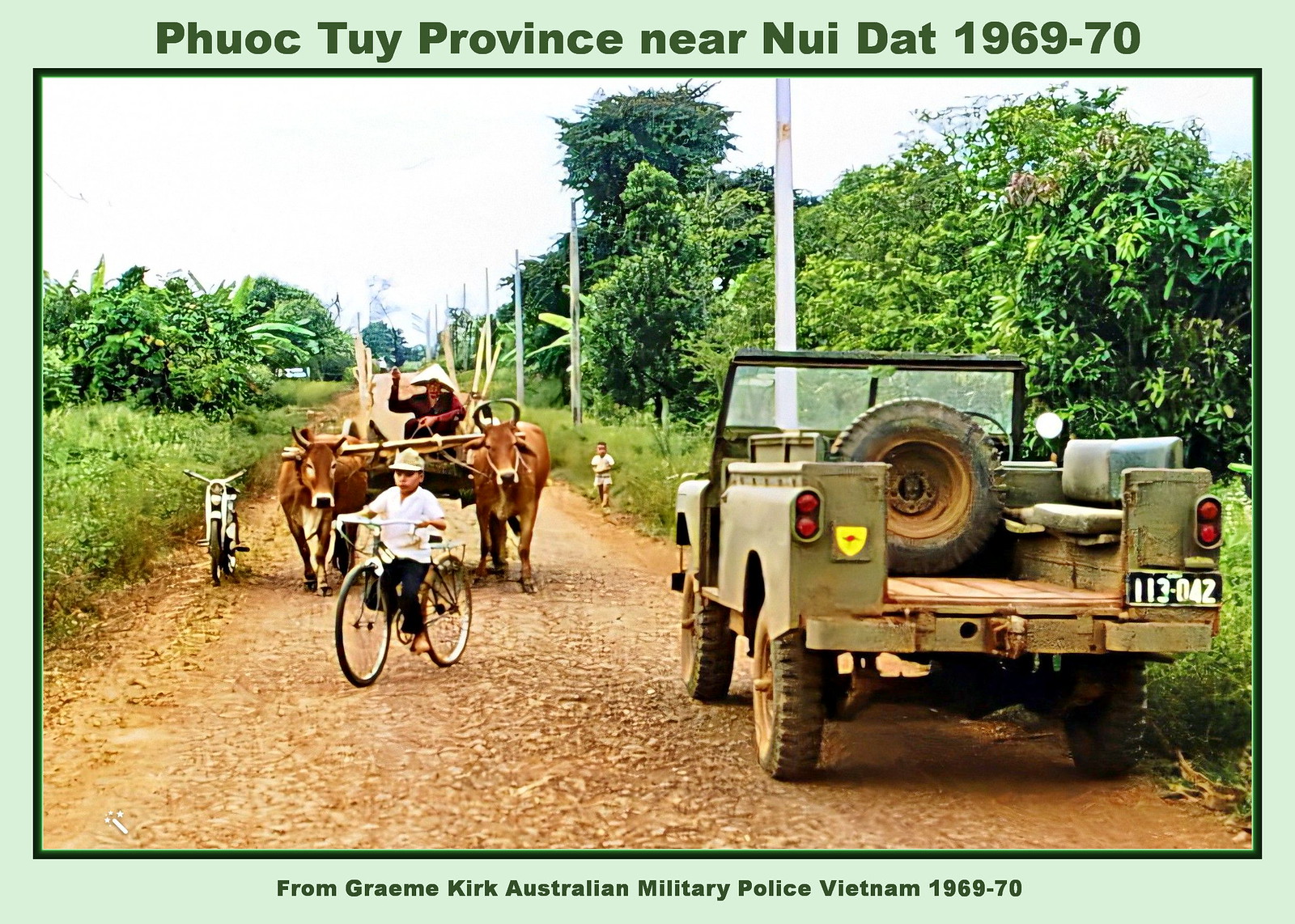In this full-color daytime photograph from Vietnam, dated 1969-1970, a reddish-brown dirt road stretches into the distance, flanked by tall grass and trees. On the right side of the road, a military jeep painted dark green or brown with the license plate 113-042 is parked, its empty pickup bed hinting at its readiness to transport soldiers. Moving along the road, a small boy dressed in white pedals a bicycle, leading the scene. Behind him, a traditional cart, drawn by two brown oxen and carrying a man in a conical hat who waves at the cameraman, adds a historical rural touch. A parked motorcycle appears on the right edge of the road. In the far background, another young boy, dressed in white, stands by the roadside, next to the series of evenly spaced white poles lining the right side of the road. The photograph is set against a washed-out sky, indicating bright, perhaps oppressive, sunlight. Encased in a light green digital frame with dark green text, the image is labeled "Phuoc Tuy, near Nui Dat, 1969-70" at the top, and credits "Graham Kirk, Australian Military Police, Vietnam, 1969-70" at the bottom.